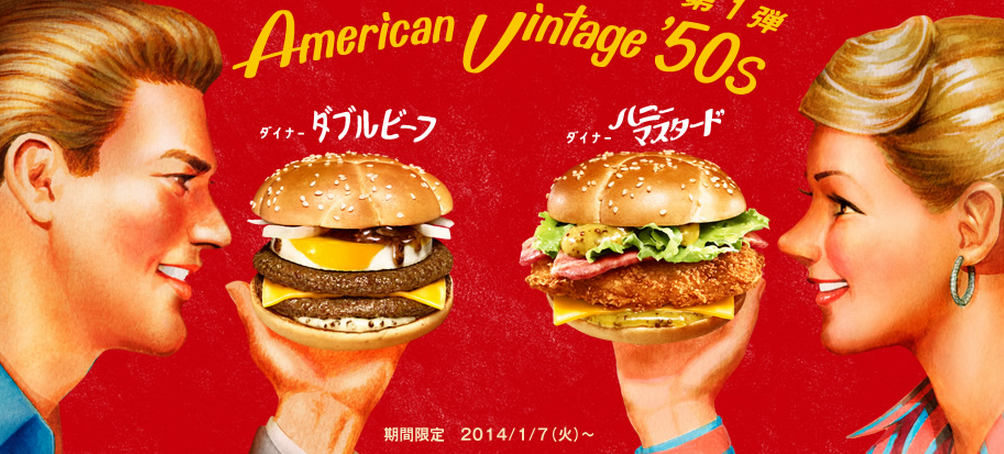This vibrant advertisement, reminiscent of a vintage 1950s style, showcases a cheerful, animated couple against a bold red backdrop. The ad, potentially for a billboard, draws attention with the headline "American Vintage 1950s" in striking yellow text. The left side features a young, smiling man with blonde, combed-back hair, dressed in blue. He holds a realistic double beef patty burger with sliced onions, a fried egg, and barbecue sauce. Facing him on the right is a young woman with blonde hair, adorned with earrings and wearing a blue and orange collared shirt. She holds a visually authentic fried chicken sandwich with lettuce and bacon. Above each sandwich, there are Japanese characters, adding an international flair. Additional Japanese text at the bottom includes the date "2014/1/7," suggesting the ad promotes a vintage American-style burger experience released in early 2014.